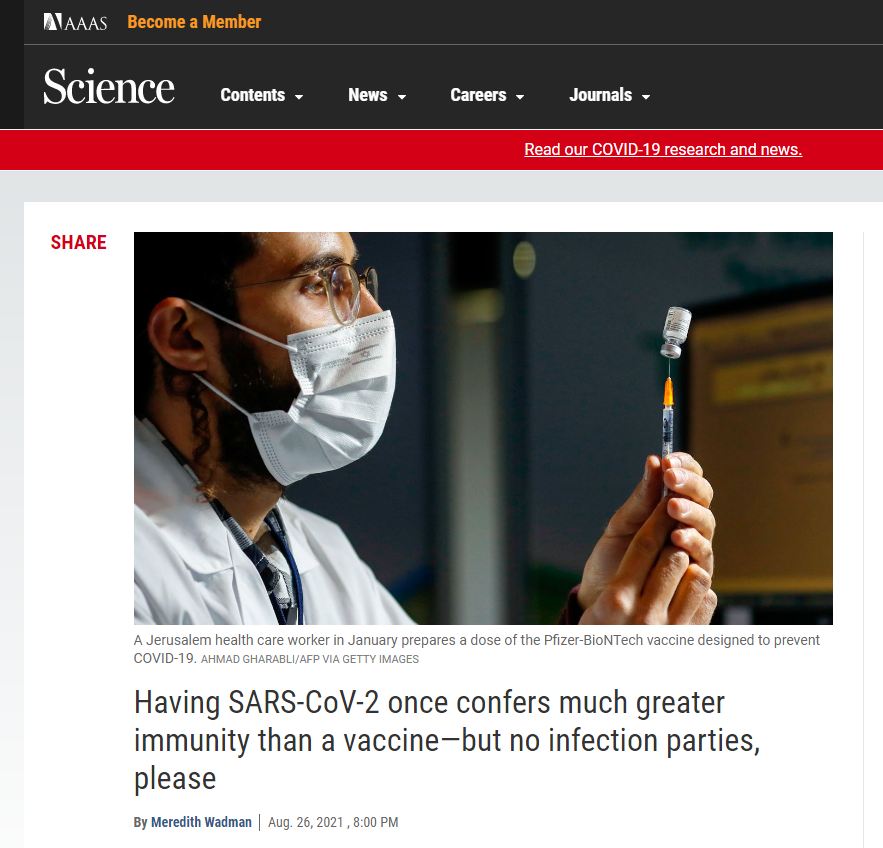The screen capture prominently displays information related to COVID-19 research, framed by a clean, professional layout. At the top, there's a black bar containing the text "AAAS," accompanied by a small square icon. To the right, in vibrant orange, is the call to action "Become a Member."

Moving downward, we see the white text "Science" followed by multiple dropdown options labeled "Contents," "News," "Careers," and "Journals." Below this is a bold red band featuring an important notice in white: "Read our COVID-19 research and news."

Further down, there's a red "Share" button, followed by an image of a healthcare worker. The individual, who has brown skin and wears glasses and a white face mask, exhibits defined facial hair and a noticeable curl of brown hair peeking from behind the ear. The healthcare worker is handling a vial and a syringe, which has an orange cap covering the needle.

Accompanying the image is a gray caption: "A Jerusalem healthcare worker in January prepares a dose of the Pfizer-BioNTech vaccine designed to prevent COVID-19." The photo is credited to Ahmad Gabol AFP via Getty Images.

Below this, a headline in black-gray text states: "Having SARS-CoV-2 once confers much greater immunity than the vaccine but no infection parties, please." Authored by Meredith Wadman, whose name appears in blue, the article is dated August 26, 2021, at 8 p.m., with the date appearing in a gray-black hue.